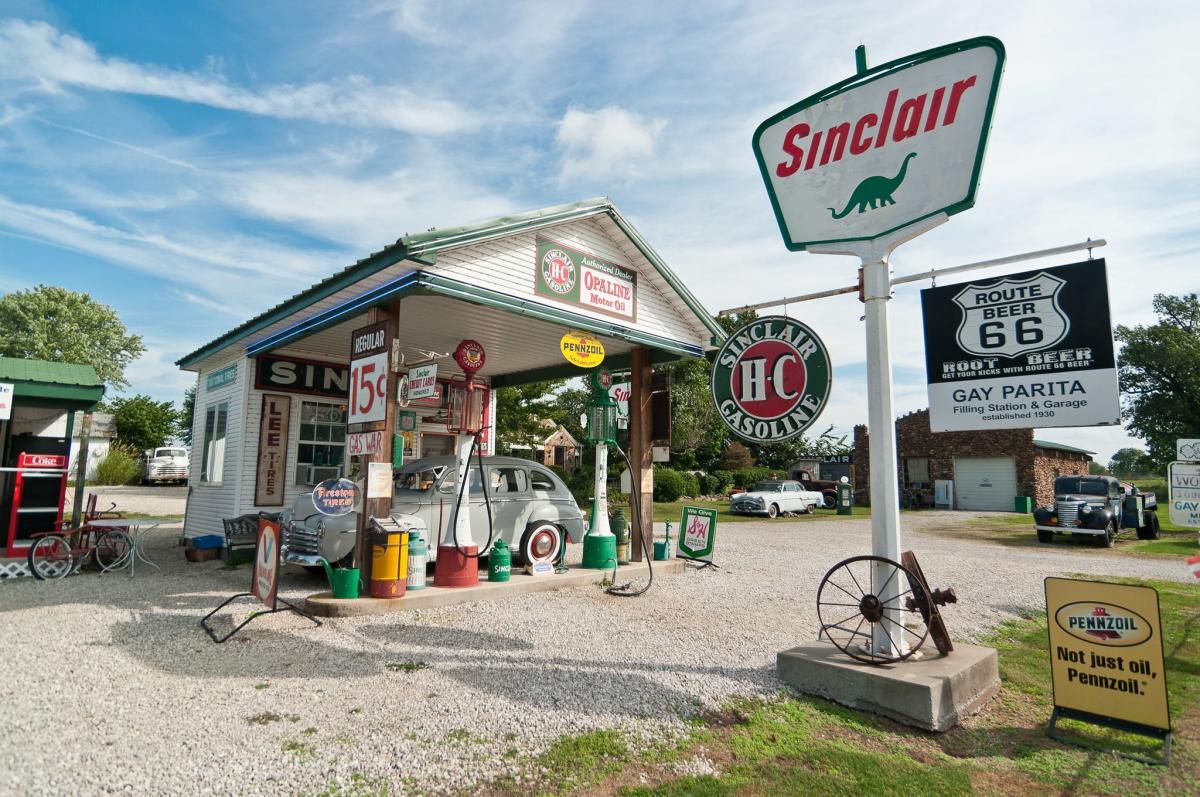The image is a color photograph of a nostalgic, old-fashioned Sinclair gas station, decorated with numerous vintage signs and details, likely situated along the famous Route 66. A distinctive white post with green borders prominently displays the Sinclair name in red letters, accompanied by the trademark green dinosaur logo. Adjacent signage mentions Route 66 and promotes various products like Route 66 Beer and Pennzoil. The station itself, labeled as Gabe Parita Filling Station and Garage, established in 1930, features an overhang sheltering exceptionally old gasoline pumps with glass tanks on top. There are hoses for filling tanks and an antique gray car parked at the pump. Antique trucks and cars, dating from the 1930s to the 1960s, are visible around the station, adding to the vintage feel. The plot of land around the gas station includes a gravel parking lot and patches of grass, set against a backdrop of a clear blue sky with scattered clouds. A sign at the pump humorously advertises gas at $0.15 per gallon, further enhancing the sense of a meticulously recreated museum display commemorating bygone eras.